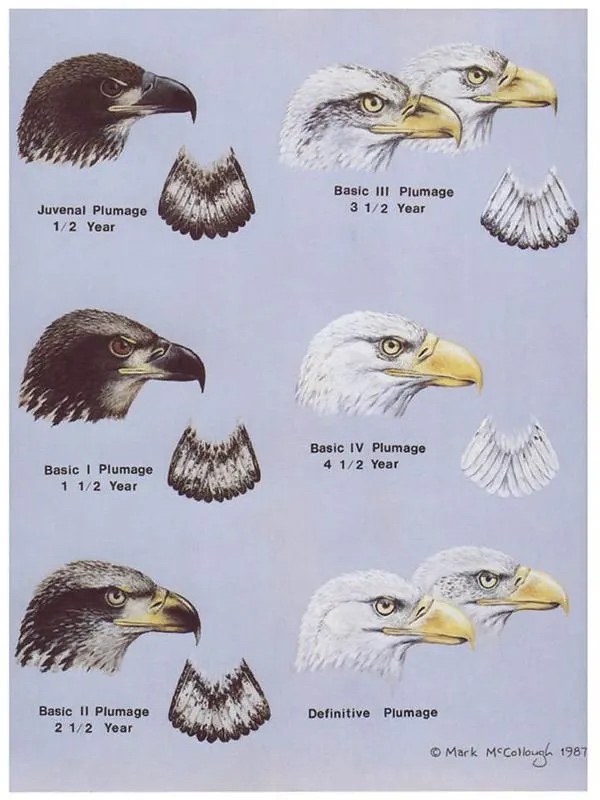This detailed image is a pedagogical poster illustrating the progression of an eagle’s plumage through different stages of its maturity. The left side of the poster showcases various eagles with predominantly black plumage transitioning from juvenile to maturity, each with distinct eye and beak colors. The eagles are carefully drawn, featuring heads with black feathers and brown eyes initially, which gradually become lighter, culminating in yellow eyes. The beaks also vary from black to gray to yellow as they mature. The plumage is depicted as black with nuanced white interiors, emphasizing changes in feather patterns.

Adjacent to it on the right side, the eagles exhibit white plumage, maintaining consistent yellow beaks and uniform eye color. The variations lie in the shading of their head feathers: the top ones have more gray, the middle ones less so, and the bottom ones almost none, indicating the progression to fully white plumage.

Additionally, a detailed schematic on the right side specifies the stages of plumage development: starting with "juvenile plumage" at half a year old, progressing through to "basic one plumage" at one and a half years, and so on until "basic four plumage" at four and a half years, each marked by distinctive changes in color and feather patterns. The final stage, labeled "definitive plumage," displays eagles with fully white heads and yellow beaks. Each stage is accompanied by drawings of eagle heads, detailing the progressive reduction of brown feathers and increase in white feathers and beak color transformation from black to yellow. Notably, the bottom right corner of the image is signed by the artist, Mark McCullough, dated 1987.